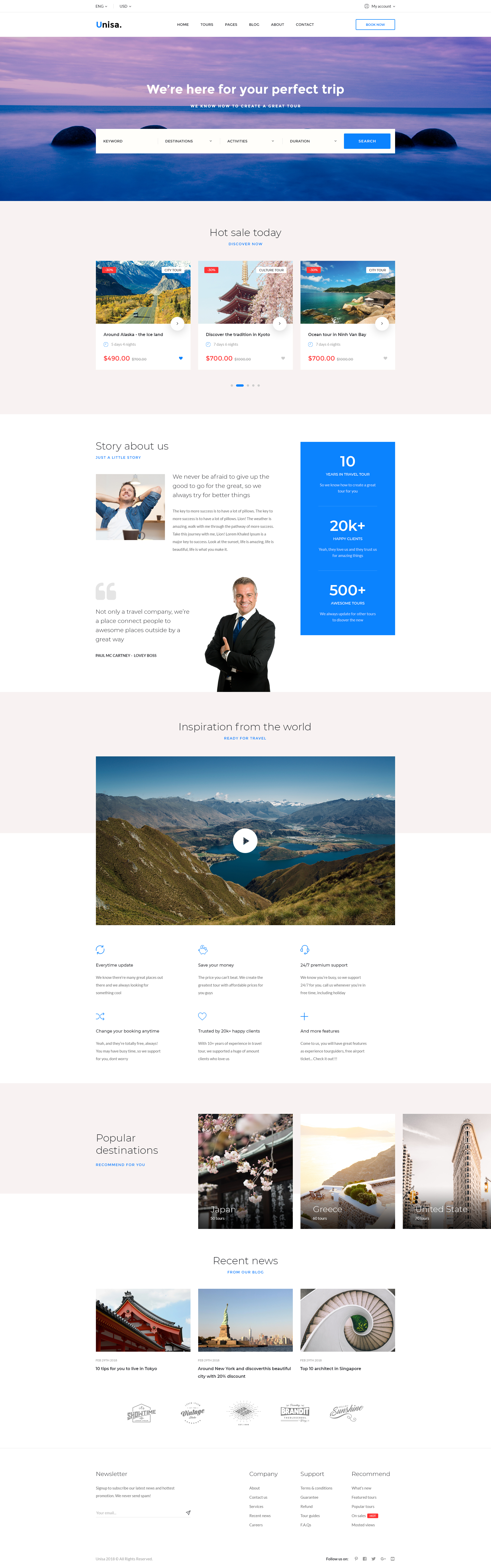**Screenshot: Detailed Description of a Travel Agency Web Page**

The screenshot depicts a travel agency's web page with a user-friendly interface. 

- **Top Navigation:**
  - In the upper left corner, the options to select "English" and "USD" through drop-down menus are available.
  - The upper right corner features a "My Account" section, also accompanied by a drop-down menu.

- **Main Navigation Bar:**
  - Positioned under the top navigation, aligned on the left side, is the site logo displaying "UNISA."
  - The navigation bar stretches across the screen from left to right with the following menu items: Home, Tours, Pages, Blog, About, Contact, and Book Now.

- **Hero Section:**
  - Below the main navigation is a prominent banner—a large rectangle filled with an aesthetically pleasing gradient of purple and blue hues, evoking the image of clouds on the horizon above a sea.
  - Overlaid text in white reads "We're here for your perfect trip," followed by the subtitle "We know how to create a great tour."
  - Nestled within this banner is a white rectangle containing interactive search options: Keyword, Destinations (with a drop-down menu), Activities (with a drop-down menu), Duration (with a drop-down menu), and a Search button.

- **Promotional Section:**
  - Beneath the banner, a promotional area highlights current offers with the heading "Hot Sale Today, Discover Now."
  - Tour packages displayed include:
    - "Around Alaska" priced at $490 for 5 days and 4 nights.
    - "Discover the Traditional in Kyoto" priced at $700 for 7 days and 6 nights.
    - "Ocean Tour in Ninh Banh Bay" also priced at $700 for 7 days and 6 nights.

- **About Us Section:**
  - A narrative follows this promotional section with an inspiring message:
    - "We never be afraid to give up the good to go for the great. So we always try for better things. The key to more success is to have a lot of pillows."
    - Interspersed with seemingly motivational quotes: "Lion, the weather is amazing. Walk with me through the pathway of more success. Take this journey with me, Lion."
    - It concludes with an uplifting note: "Not only a travel company, we're a place that connects people to awesome places outside by a great way" and a callout to "Paul McCartney, lovely boss."
    - The section asserts their credibility with "Ten years in travel tour so we know how to create a great tour for you," "20,000+ happy clients," and "500+ awesome tours and inspiration from the world."

- **Visual Section:**
  - Below this text is an accompanying image of mountains and a serene lake. 

- **Popular Destinations:**
  - The web page lists popular destinations such as Japan, Greece, and the United States.

Each element is designed to convey reliability and inspiration, guiding the user smoothly through their travel planning experience.